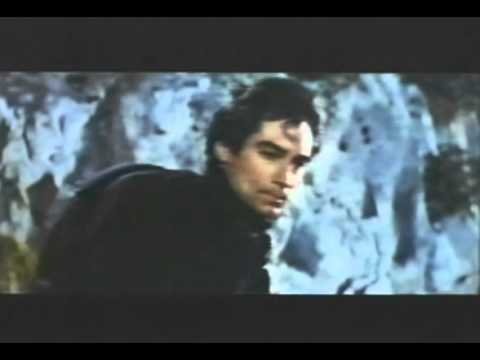The image is a low-quality, washed-out movie still that appears to have been taken from an older, possibly VHS format. It features a man of possibly Greek or Middle Eastern descent, characterized by his very tan complexion, chiseled face, thick dark eyebrows, and dark wavy hair that reaches his ears, with a distinctive curly strand hanging on his forehead. Dressed in a black turtleneck or high-collar jacket that reaches up to his chin, he looks downwards with a slightly agitated or pensive expression. The background showcases white, snowy mountains or a craggy, rocky landscape. The screen is framed by dark widescreen bars at the top and bottom, with the image being viewed from the man’s mid-chest upwards.